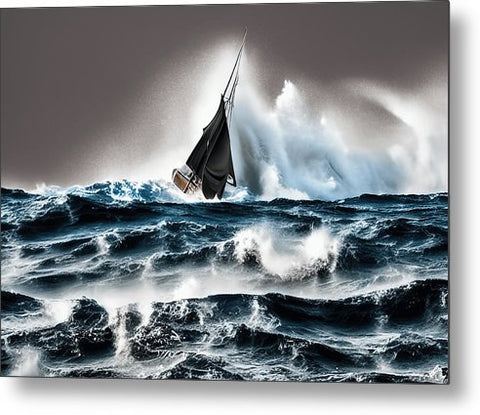The image depicts a highly detailed realistic painting, likely generated, of a small sailboat struggling in an angry, stormy sea. The turbulent navy blue ocean features tall, frothy waves with white caps, and massive splashes of water shoot upwards, almost engulfing the vessel. The sailboat, which is positioned towards the middle and slightly to the back of the scene, has a black sail that appears to be falling off, adding to the sense of distress. The front of the boat is submerged under the powerful waves, emphasizing its fight against the elements. The sky is a dark, ominous gray, contrasting sharply with the light around the boat caused by the white spray of the crashing waves. This artistic portrayal captures the ferocity and chaos of the stormy sea, making the sailboat seem minuscule and vulnerable amidst the vast and tumultuous ocean.